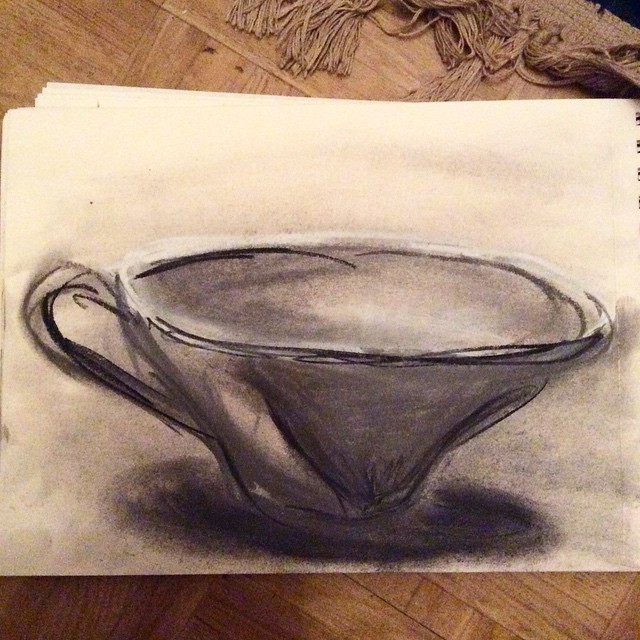In this photograph, we see an artistic, heavily shaded illustration of a small teacup, likely drawn with charcoal or a pencil, centered on a white piece of paper. The teacup features a tall arch from the bottom to the top, a thick rim, and a curved handle extending to the left. The drawing includes detailed shading, creating a pronounced shadow beneath the cup and additional blended shadings in the background. This central sheet of paper is placed atop several other fanned-out sheets, all situated on a wood-finished tabletop. In the top right corner of the image, there are decorative fringe-like tassels, possibly from a woven object, adding an extra element of texture to the scene.